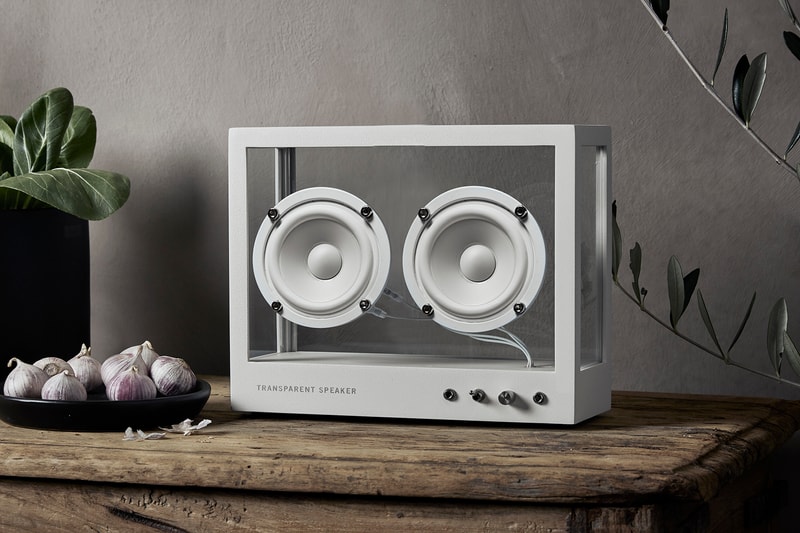In the image, we see a detailed scene featuring a distressed, old wooden table, likely made of oak and unvarnished. Dominating the center is a large, attractive white audio speaker encased in a transparent box with visible internal components, including two floating audio speakers with paper cones. The box is labeled "Transparent Speaker" in small capital letters at the bottom. Below the speaker are four knobs, and possibly two audio inputs with some visible wiring.

To the left of the speaker, there is a black dish containing cloves of garlic. Further left, partially visible, is a tall black planter with a green leafy plant that might be lettuce or cabbage. On the right side of the speaker, some sprigs with long, spindly branches and pairs of leaves emerge into the frame. The background features a textured gray wall, enhancing the muted top-left light source that subtly illuminates the scene, giving it an artistic and slightly surreal vibe, reminiscent of a computer-generated or AI-created image.